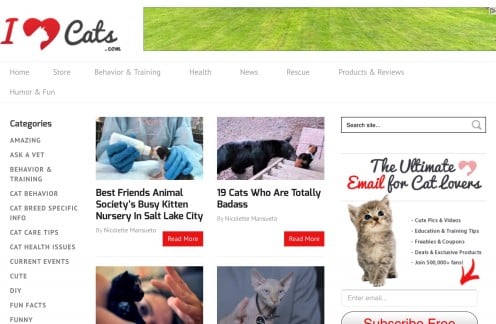This is a detailed screenshot of the website ilovecats.com. The website header features the text "I Love Cats" where the "I" is red, "Love" is represented by a heart containing a white cat silhouette, and "Cats" is written in black cursive. At the very top, there is a green and yellow banner.

Below the banner, there is a navigation menu with the following categories: Home, Store, Behavior and Training, Health, News, Rescue, Products and Reviews, and Humor and Fun. The main content area showcases four articles, each accompanied by images and red "Read More" buttons. The first article is titled "Best Friends Animal Society's Busy Kitten Nursery in Salt Lake City," and the second article is titled "19 Cats Who Are Totally Badass."

On the left side of the page, there is a categorized list including: Amazing, Ask a Vet, Behavior and Training, Cat Behavior, Cat Breed Specific Info, Cat Care Tips, Cat Health Issues, Current Events, Cute, DIY, Fun Facts, and Funny.

A search bar with the placeholder text "Search site" is also present for easy navigation. Additionally, there is a promotional section featuring a picture of a kitten with the title "The Ultimate Email for Cat Lovers." Below this, there is a subscription form to enter your email address, along with a button labeled "Subscribe Free." The section promotes receiving cat-related content including cute pics and videos, education and training tips, freebies and coupons, deals, and fantastic products. Members are encouraged to join, as indicated by the phrase "Join with [number]."